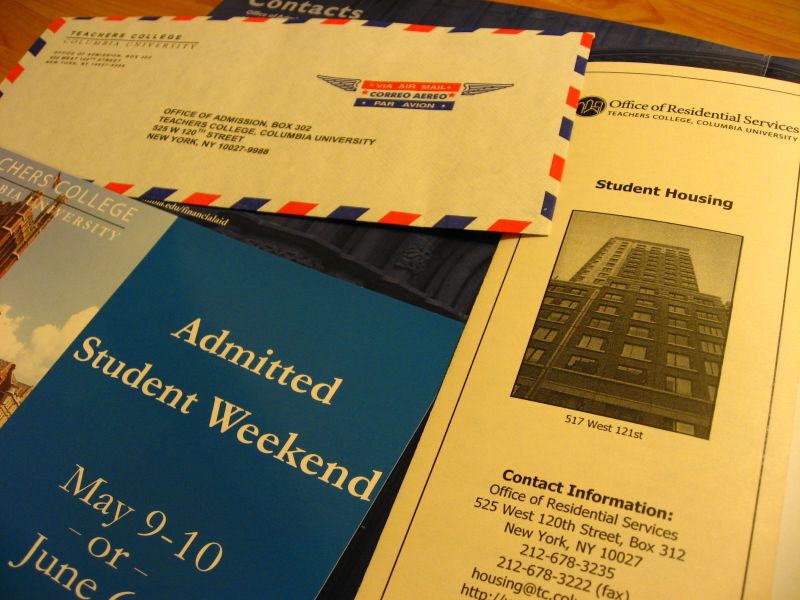In this detailed photographic image, a wooden table serves as the backdrop for a collection of mail and brochures. At the center, an envelope marked with a distinct red, white, and blue border and a matching logo prominently states "Via Air Mail" in red, "Correo Aéreo" in white, and "Par Avion" in blue, with wing designs on the sides. Addressed to the Office of Admissions, Box 302, Teachers College, Columbia University, 525 West 120th Street, New York, NY 10027-9986, this envelope catches the eye.

To the left of the envelope is a blue brochure, with tan writing announcing "Admitted Student Weekend, May 9-10 or June," accompanied by an image of the college building.

On the right side, a black and white brochure heads the "Office of Residential Services, Teachers College, Columbia University, Student Housing," featuring a high-rise building. This brochure provides contact information for the Office of Residential Services at 525 West 120th Street, Box 312, New York, NY, and lists phone numbers 212-678-3235 and 212-678-3222.

Together, these pieces of mail and brochures, set against the wooden table, paint a detailed picture of communications from Teachers College, Columbia University, encompassing admissions, student housing, and upcoming events for newly admitted students.